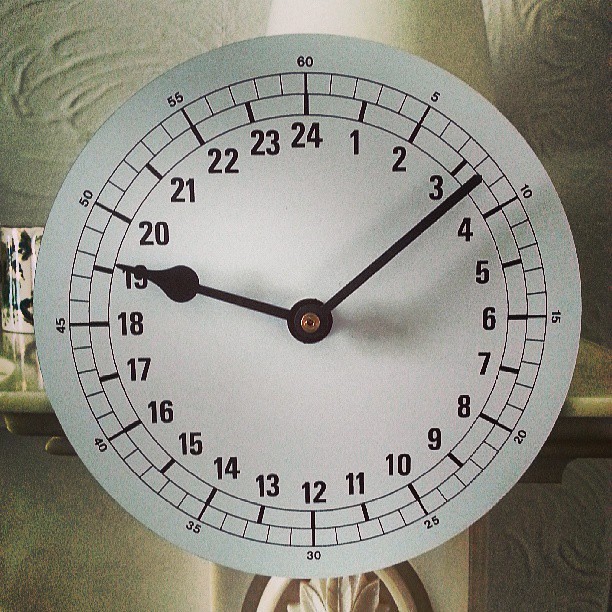This color photograph captures a close-up of a homemade 24-hour clock, meticulously crafted from white paper. The circular clock face features a dual-layer numbering system. The inner layer displays hours from 1 to 24, while the outer layer is marked with minutes in intervals of five, ranging from 5 to 60. Both sets of numbers are printed in black, creating a stark contrast against the white background. The black hour and minute hands, appearing to be made from paper and fastened at the center, currently indicate approximately 13 minutes past 1900 hours. Behind the clock, the backdrop consists of bunched-up white fabric or paper towels, with the lower section of the image revealing a soap package adorned with a flower. The overall setting presents an unassuming yet detailed representation of a handmade 24-hour clock against a simple, off-white background.